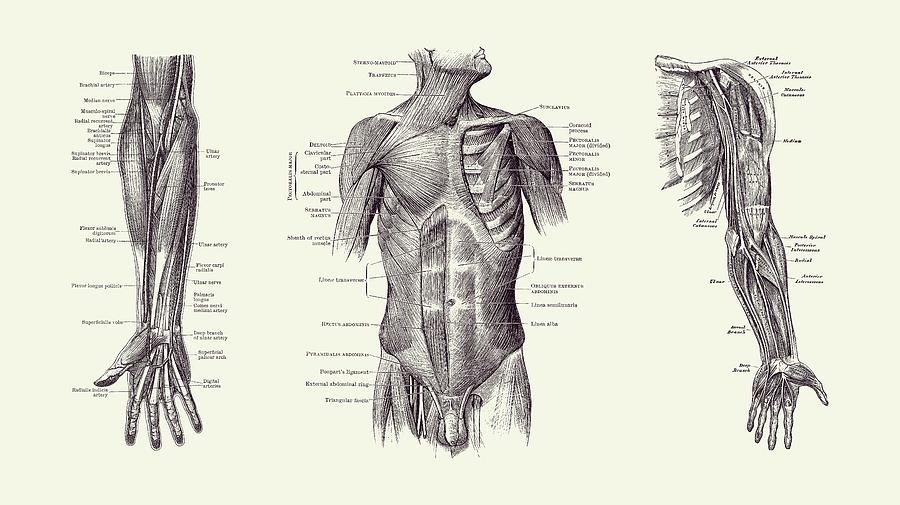The image is a detailed, horizontally oriented, rectangular illustration from a medical book, depicting a doctor's diagram of a male human body. The background is a yellowish beige color. The diagram is divided into three main sections: the left arm, the torso, and the right arm. Each section reveals a comprehensive, almost x-ray-like view of the body's internal structures, including muscles, tendons, bones, and other anatomical features. The left section shows the forearm, from just above the elbow down to the hand, with labels and arrows pointing to various muscles and tendons. The central section displays the torso, spanning from the chin down to just below the groin area, labeling the ribs, muscles, tendons, and even extending to the upper leg and penis. The right section illustrates the shoulder and arm, again with detailed annotations of muscles, tendons, and bones. Each body part is meticulously labeled with black text, though the labels are too small to read clearly in the image.